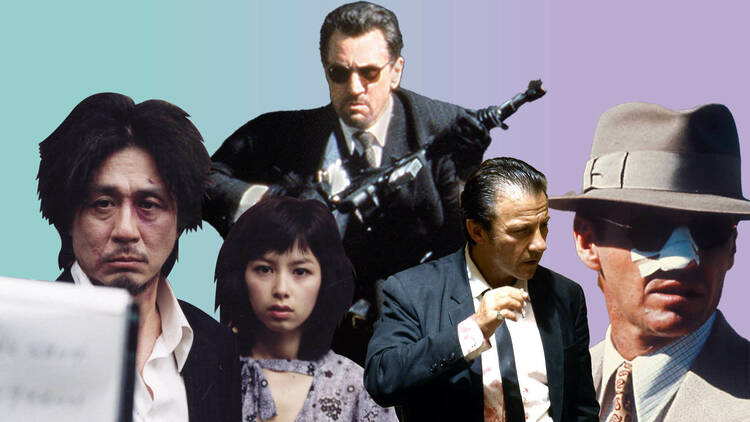The image is a collage that evokes the style of a disorganized movie poster, featuring cutouts of various film characters set against a gradient background transitioning from aqua-blue to light violet. On the far left is a mid-aged Asian male, likely the protagonist from Oldboy, followed by a younger Asian female. Above them is a menacing white man dressed in an expensive suit with black leather gloves and sunglasses, holding an automatic rifle—a character reminiscent of those from the film Heat. Next is another white male with dark hair, also in a suit and smoking a cigarette, which aligns with Harvey Keitel's role in Reservoir Dogs. Lastly, there is a close-up of Jack Nicholson's character from Chinatown, identifiable by his brown fedora, sunglasses, and bandaged nose. In the bottom left corner, a blurry notepad is partially visible, though its contents are unreadable.